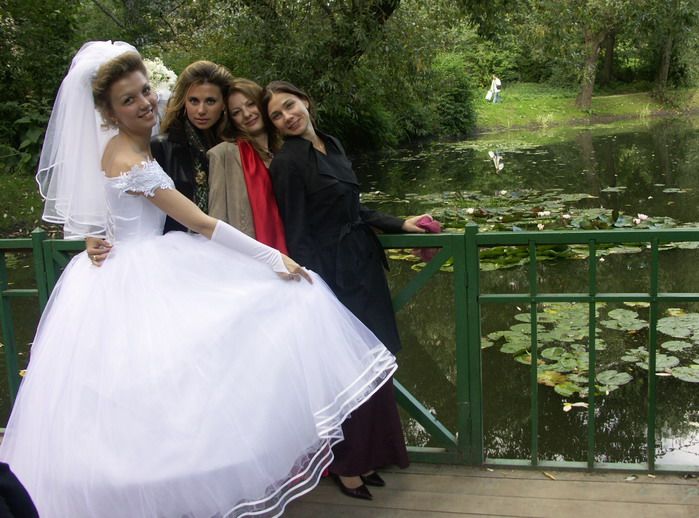In this photograph, four women are standing together outdoors in front of a green metal fence and gate, with a picturesque pond behind them, featuring lily pads growing in two distinct sections. The backdrop includes lush green grass and trees. From left to right, the first woman is dressed in a bridal gown with short sleeves, complemented by a veil and long white gloves. She has light brown hair pulled back. The second woman wears a dark blouse with her long hair partially pulled back. The third woman sports a beige jacket over a red satin dress, with her long light brown hair cascading down. The fourth woman is clad in a black overcoat and a long skirt, holding a pink item, potentially clothing, in her left hand. They are all standing on a wooden pathway, with a visible person dressed in white walking on a path in the background near the edge of the pond.